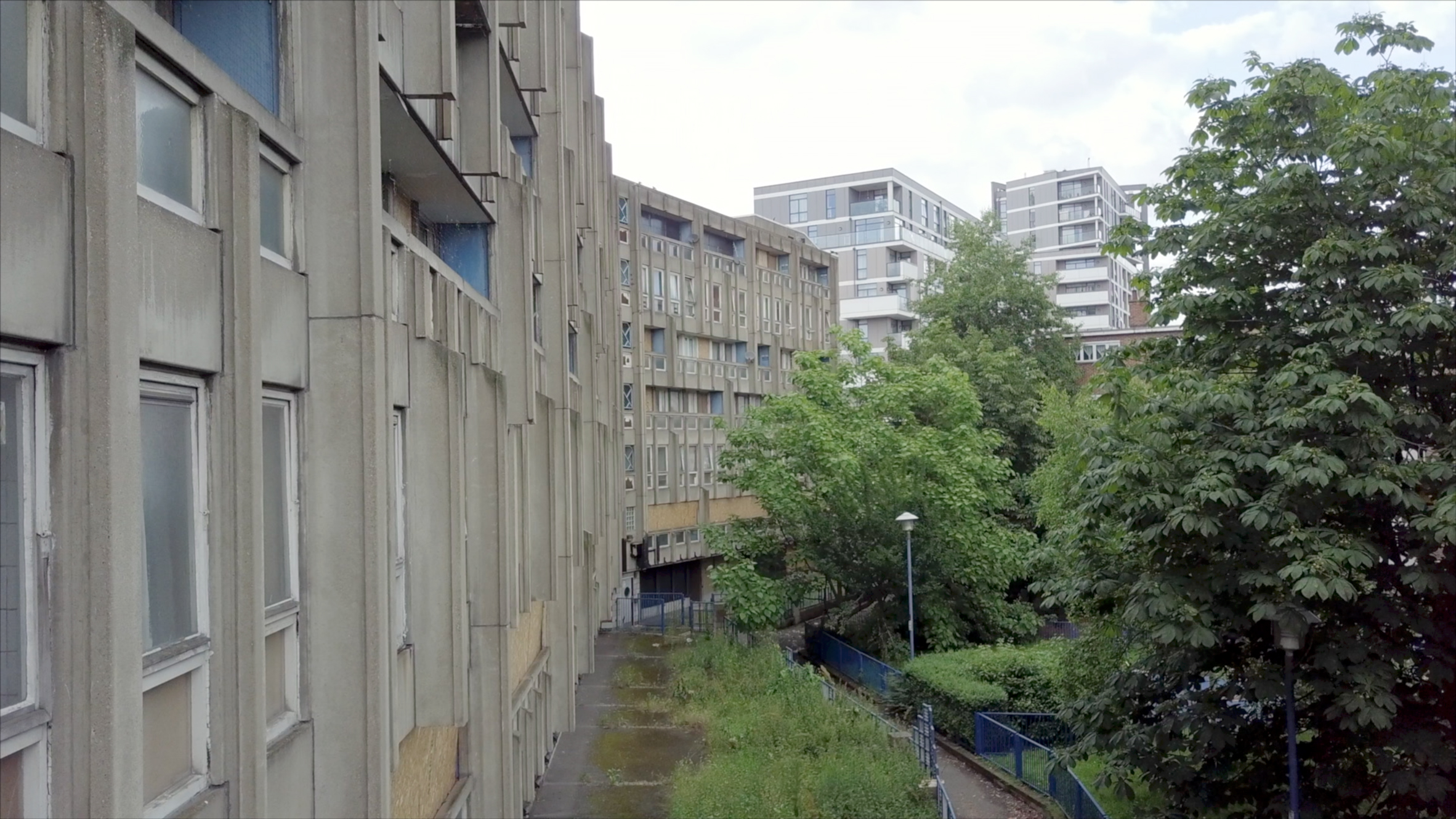The photograph depicts a slightly weathered, multi-story, gray concrete apartment building with numerous single-pane windows set into white frames and occasional yellow decorative accents on the first floor. This rectangular building extends along the left side of the image, contrasted against a backdrop of an overcast white-blue sky. Flanking the right side of the image is a lush, green-leaved tree, and below, there is a pedestrian walkway bordered by a manicured green space with grass and shrubbery. This walkway is highlighted by a blue-painted railing and a nearby light post, suggesting a communal area designed for the building's residents. The overall ambiance indicates a typical, though somewhat dated urban living environment, imbued with a sense of wear from the passage of time.